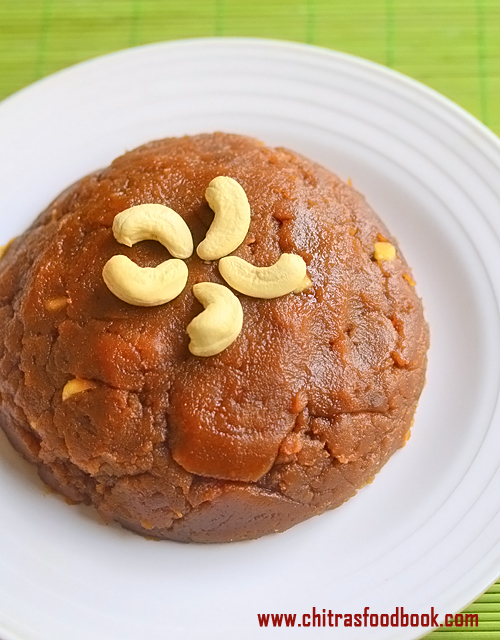The food photograph features a strikingly clear and detailed image set against a green, slightly blurry background that appears to resemble a checkered tablecloth. Dominating the composition is a pristine, circular white plate, centrally positioned to showcase the delectable focal point: a steamed pudding. The pudding, with its smooth, rounded dome shape, radiates a rich gingerbread-like hue, blending orangish and brownish tones. The top of the dessert is adorned with five cashews meticulously arranged in a circular formation, creating a star-like design at the center.

The lighting in the image comes from the right, casting a natural glisten on the pudding that highlights its moist texture, adding to its visual appeal. The overall presentation is meticulously crafted, suggesting this is a professional food blogger's work. This is further confirmed by the URL "[www.chitrasfoodbook.com](http://www.chitrasfoodbook.com)" in dark orange text placed subtly at the bottom of the image.